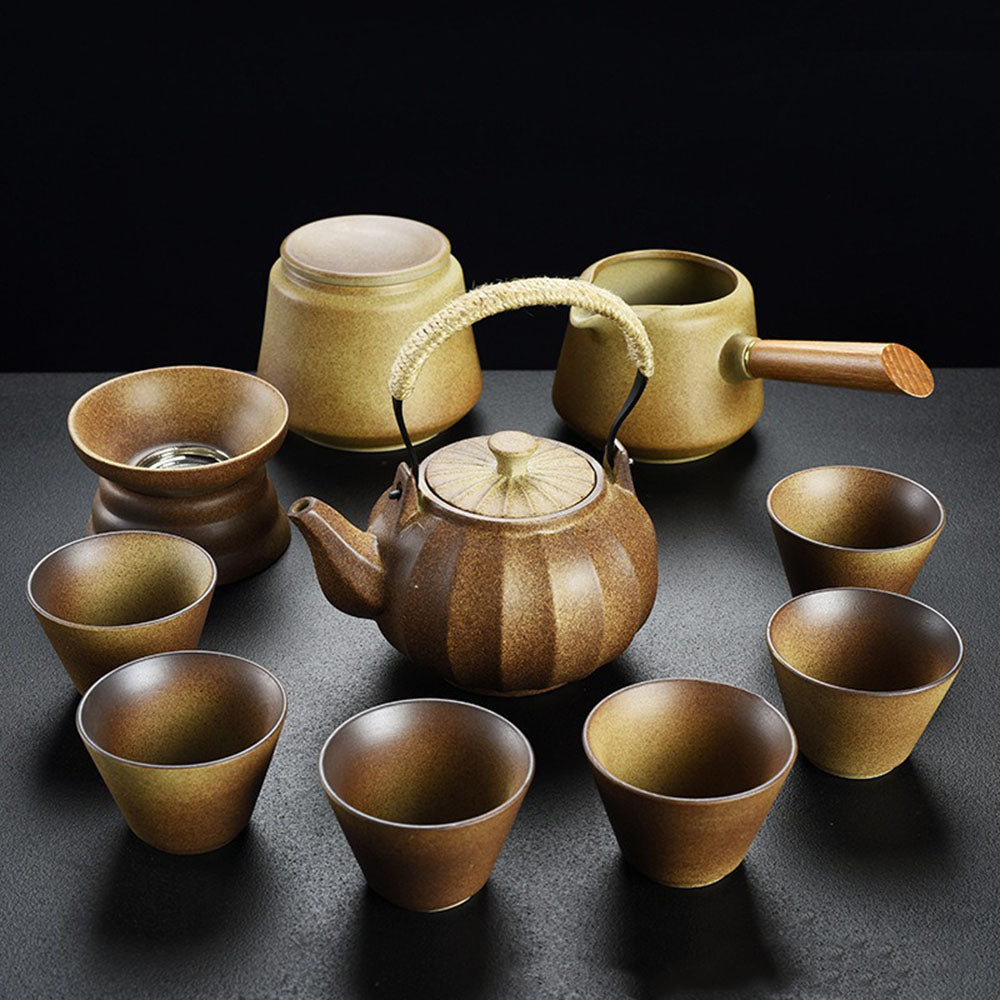In this square photograph, a collection of utensils is meticulously arranged on a dark gray surface, set against a pitch-black background that gives the image a striking contrast. At the center, a prominent brown kettle with a cream-colored lid and handle serves as the focal point. Surrounding the kettle are six light brown cups, reinforcing the cohesive color palette. Additional container utensils, including one with a distinctive wooden handle, are placed behind the kettle, contributing to the intricate composition. The overall arrangement forms a circular pattern around the kettle, creating an artistically balanced and visually appealing setup.